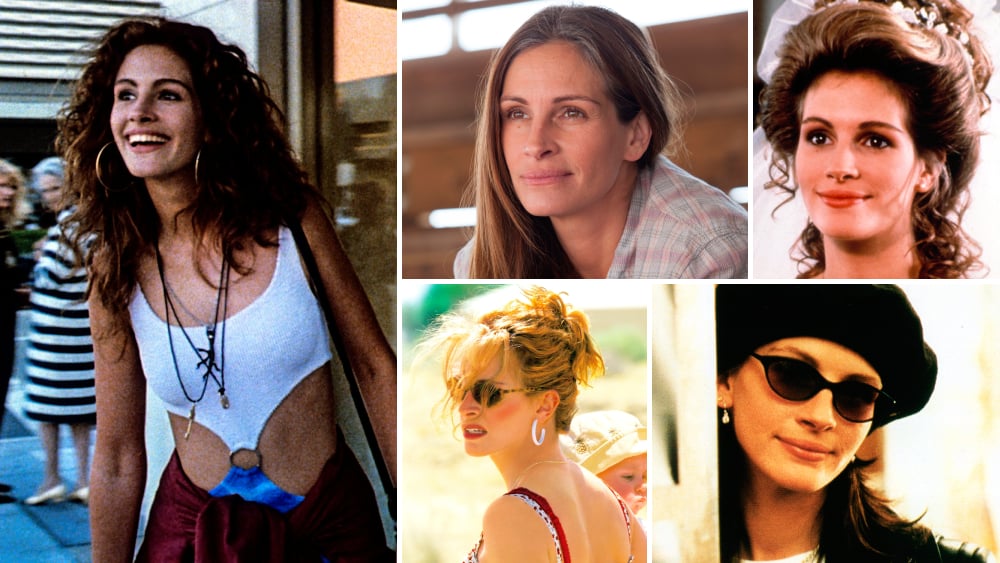This detailed collage showcases actress Julia Roberts through various stages of her career, featuring notable roles from several films. On the left, the largest and most prominent photograph captures a scene from "Pretty Woman" with Roberts smiling outdoors in her iconic outfit, while two older women on the street gaze at her with clear disapproval. To the right, four smaller images of Roberts provide a broader view of her filmography. The top center image features her with brown hair, resembling a still from "August: Osage County." Adjacent to it, on the top right, Roberts is seen seemingly dressed for a wedding, likely from "Steel Magnolias." The bottom center shot appears to be from "Erin Brockovich," showing her serious demeanor. Lastly, the bottom right image presents Roberts with a chic look, donning a black beret and sunglasses, from an unspecified film. Each photograph offers a distinct glimpse into her versatile acting career.